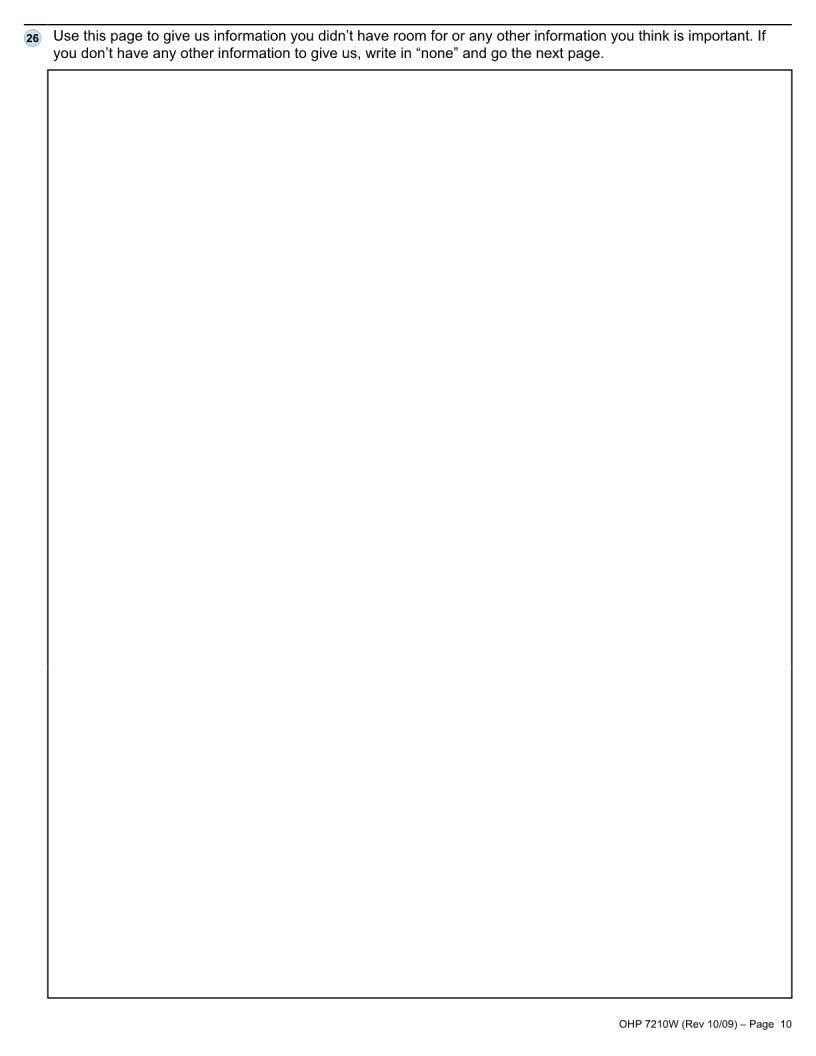The image features a prominent vertical rectangle with a black outline. Directly above this rectangle is a black line that extends slightly beyond the rectangle's length. Below this black line is a small light gray circle, containing the bolded number "26" in black. Adjacent to the circle, centered between the black line and the top edge of the rectangle, is a block of text. This text instructs viewers to "use this page to give us information you didn’t have room for, or any other information you think is important. If you don’t have any other information to give us, write in 'none' and go to the next page."

Beneath the main vertical rectangle, in the bottom-left corner of the image, is a small, light gray rectangular area that holds a brief string of text: "OHP7210W (REV1009) - Page ten" in black font. The overall layout emphasizes instructions intended for additional user-provided information.